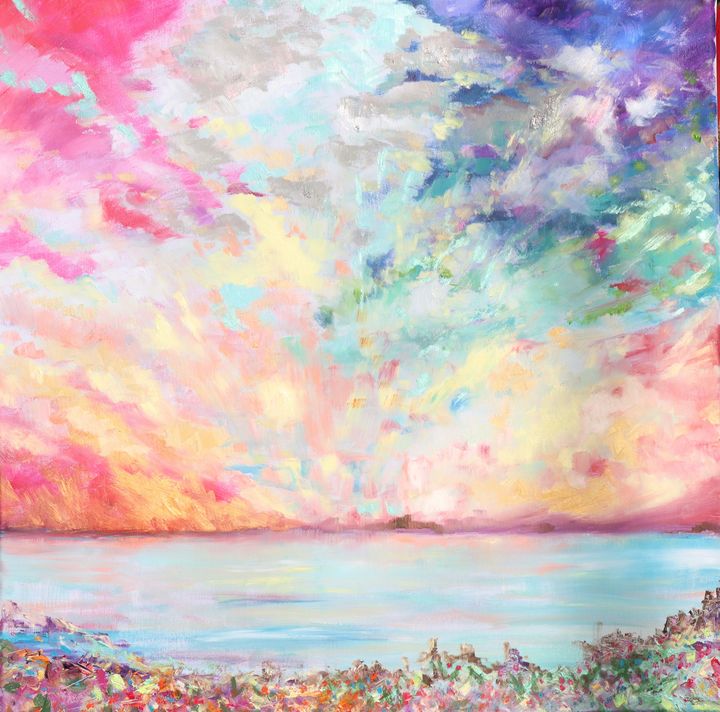The painting is a tall, abstract composition characterized by its vibrant and blended use of colors. The bottom quarter of the image is filled with water-like hues, featuring teals, light blues, and medium blues that suggest a body of water. In the foreground, an artistic interpretation of terrain showcases a mélange of greens, yellows, and pinks, with splashes of bright colors possibly representing springtime flowers. The sky is a kaleidoscope of pastel shades, transitioning from pinks, yellows, and oranges on the left and bottom to blues and greens as it ascends, culminating in purples at the upper right. The overall effect is one of a colorful, dynamic scene where the colors appear to have bled and blended together, evoking the impression of a rainbow melting and running with the rain. The painting's abstract nature leaves room for interpretation, emphasizing its bright, artistic, and beautiful aesthetic.